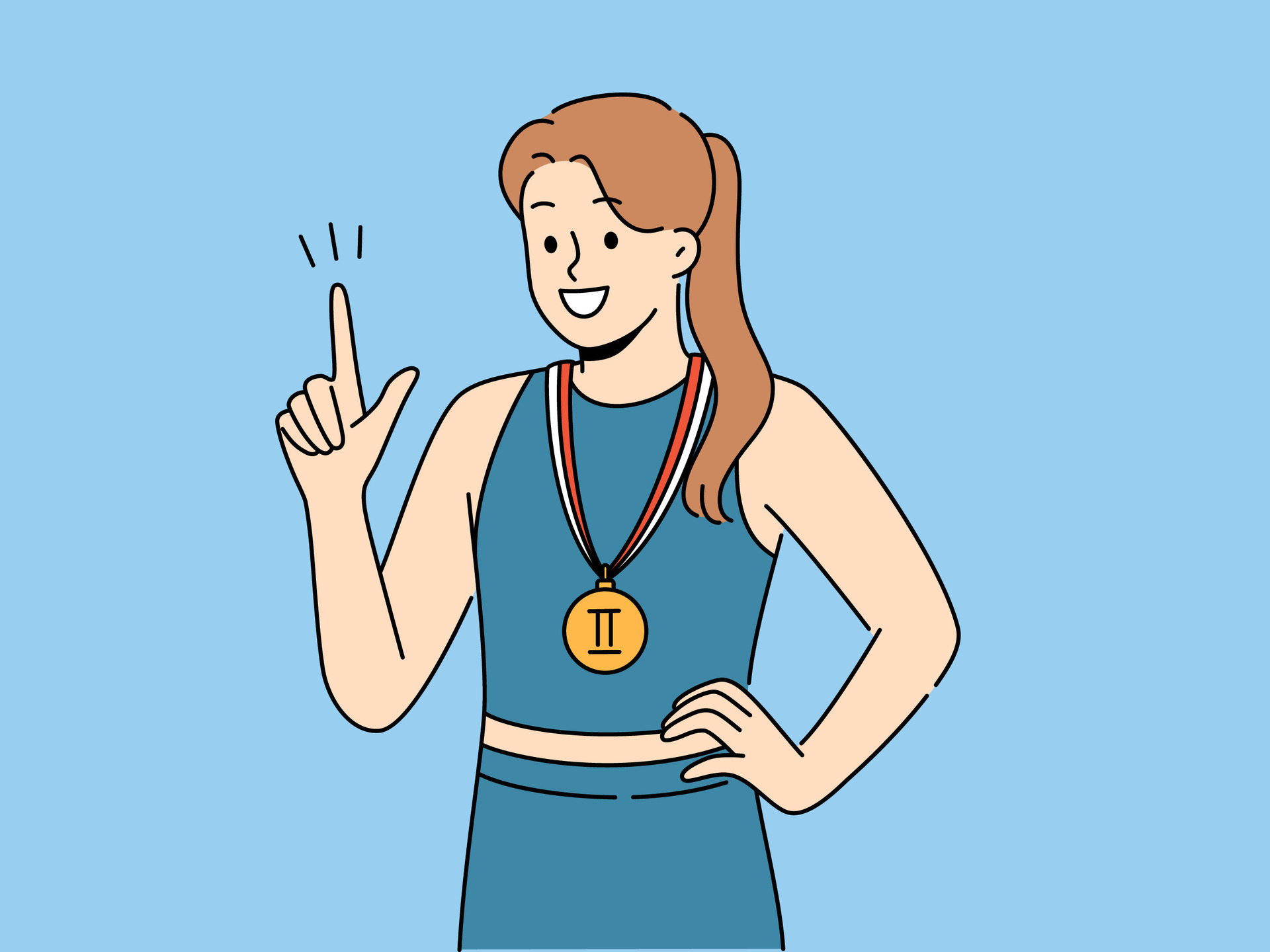This illustration depicts a young woman against an all light blue background, styled in a cartoonish manner. The woman's facial features are minimalistic, with simple black circles for eyes and a half-circle black outline for a mouth filled with white, reminiscent of old comic styles. She has long brunette hair tied in a ponytail that drapes over her left shoulder and across her front. Wearing a blue dress cinched with a white belt, the dress cuts off just below her waist. She poses confidently, her left hand resting on her hip while her right hand is raised, forming an 'L' symbol, accentuated by three small black dashes above her finger. Around her neck hangs a medal on a red, white, and blue ribbon, featuring the Roman numeral "II", suggesting a significant achievement. Her overall demeanor exudes pride and accomplishment, encapsulated in this vibrant and detailed cartoon depiction.